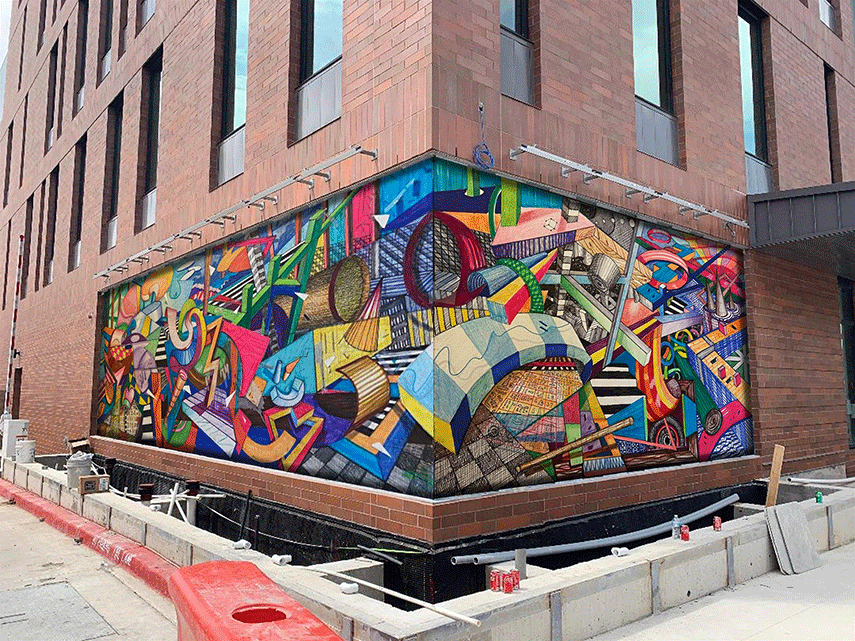The photograph captures a detailed view of a red brick building mid-construction, focusing on its corner. Prominently featured is a vibrant, abstract mural that spans the intersection of two walls, filled with various shapes and colors including blue and yellow squares, blue and white stripes with a yellow opening, and a round red shape resembling bicycle spokes. The top section of the building displays multiple stories with long narrow windows, while the bottom half showcases the colorful artwork against the red brick. A light gray cement stone barricade, accented with a red border, encircles the base, indicating ongoing construction work, including visible pipes and tools. Scattered on the cement barricade are several Coca-Cola cans, hinting at the presence of workers recently on-site. A red plastic or rubber trash can is also visible, adding to the construction-related clutter at the scene.